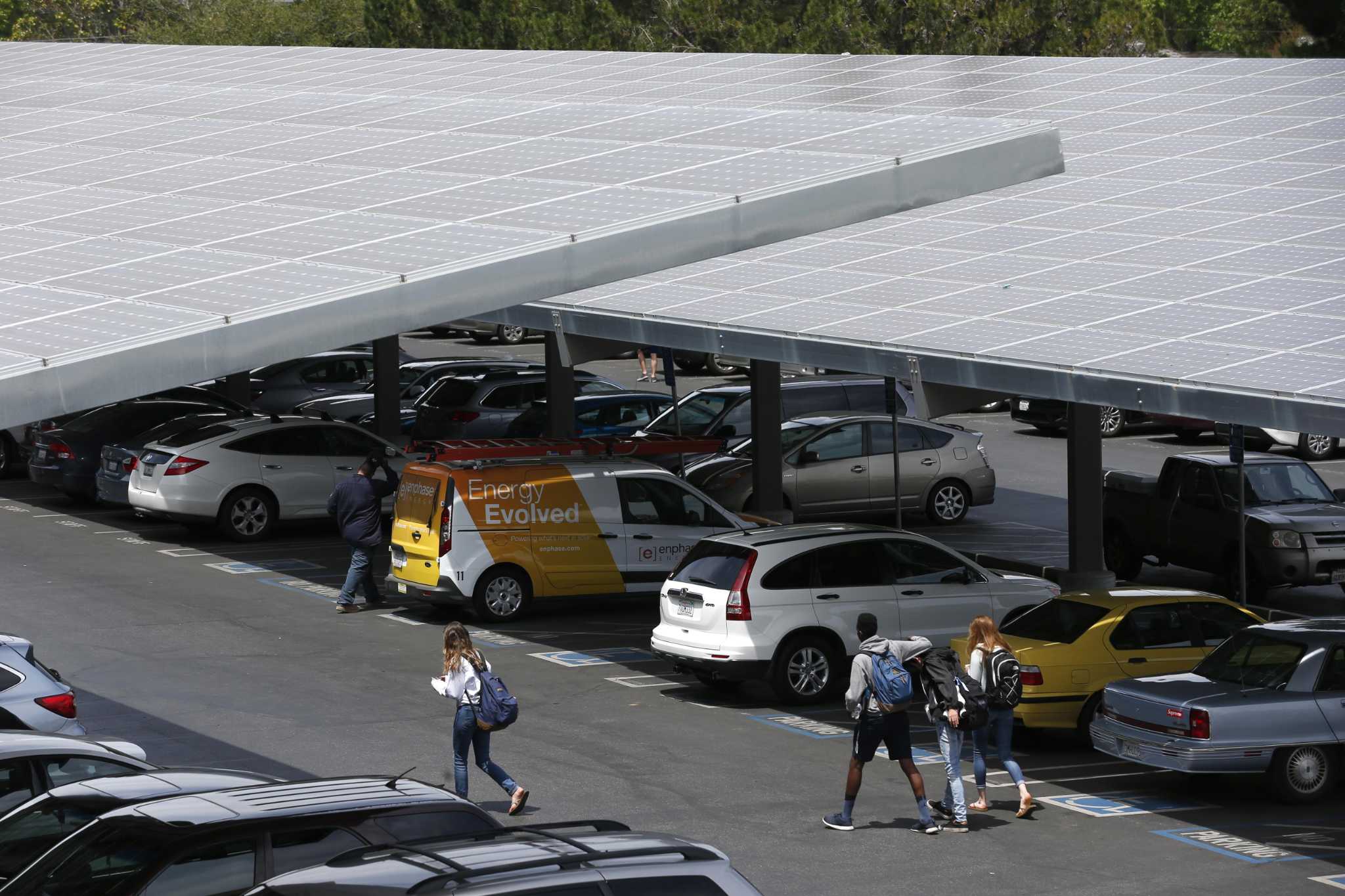This image captures the overhead view of a spacious, covered parking area, likely adjacent to an office building situated near a wooded area. The parking spaces are protected by a sloped roof made up of light gray, checked pattern panels, possibly solar panels, which are fully exposed to sunlight on this bright day. Within this scene, we see a diverse collection of vehicles, including a van labeled "Energy Evolved," suggesting potential service or installation of the solar panels. In the middle ground, four young individuals walk away from the camera down the drive aisle, dressed casually in jeans and shorts and each carrying a backpack. A notable detail is a woman on the left in a white sweatshirt and blue jeans beside a man in shorts and a white shirt, both equipped with backpacks. The background reveals the tops of green trees, enhancing the natural setting of the parking lot.